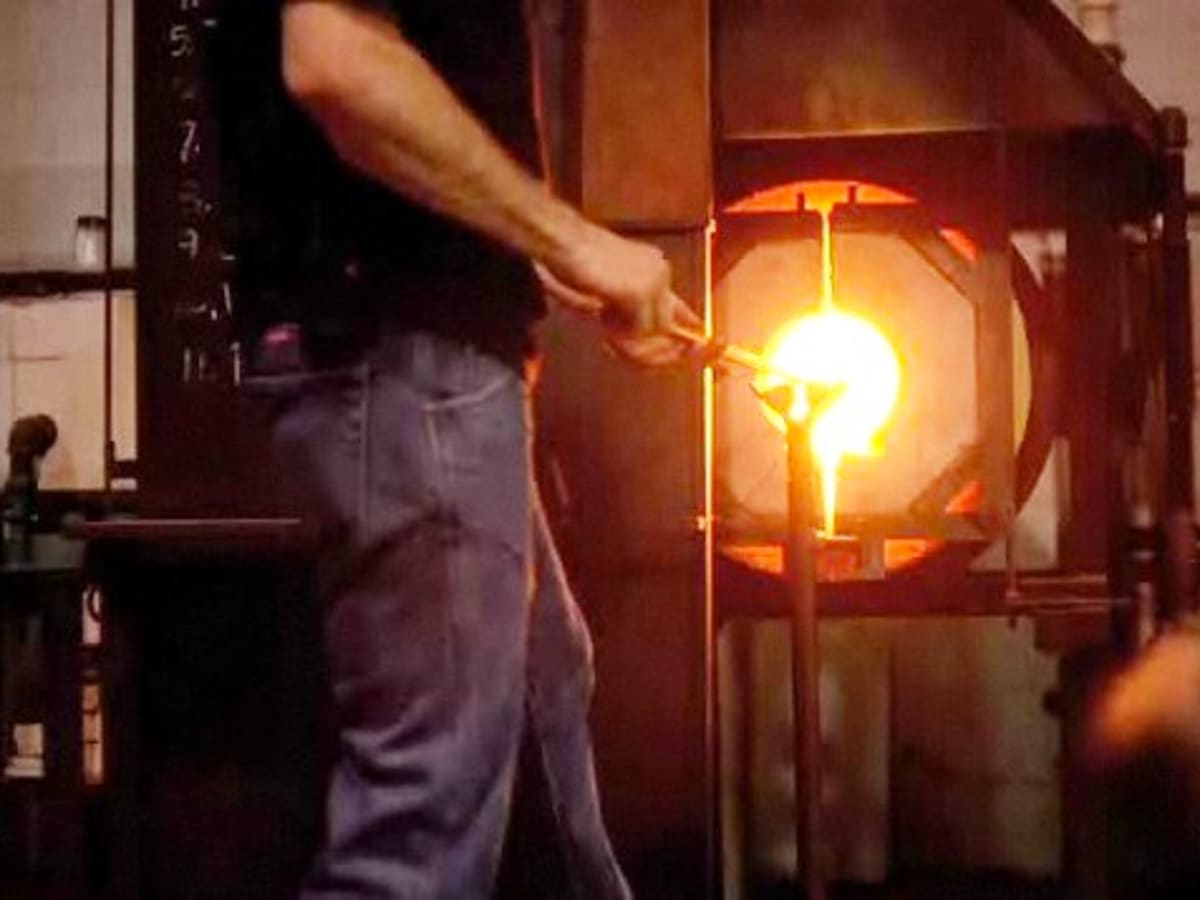The photograph, though blurry and of low resolution, depicts a man standing slightly to the left of center in what appears to be a glass-blowing studio. The man is wearing blue jeans and a black shirt. He is holding a long rod, at the end of which is a glowing, brightly colored orb emitting whitish-yellow light, suggesting he is working with molten glass. The background features various industrial elements, including metal structures, pipes, and a glass jar on a shelf. The scene is lit with an orange hue, creating shadows against the walls. The overall setting is indoors, filled with the equipment typical of glass-making or metal-smelting activities.